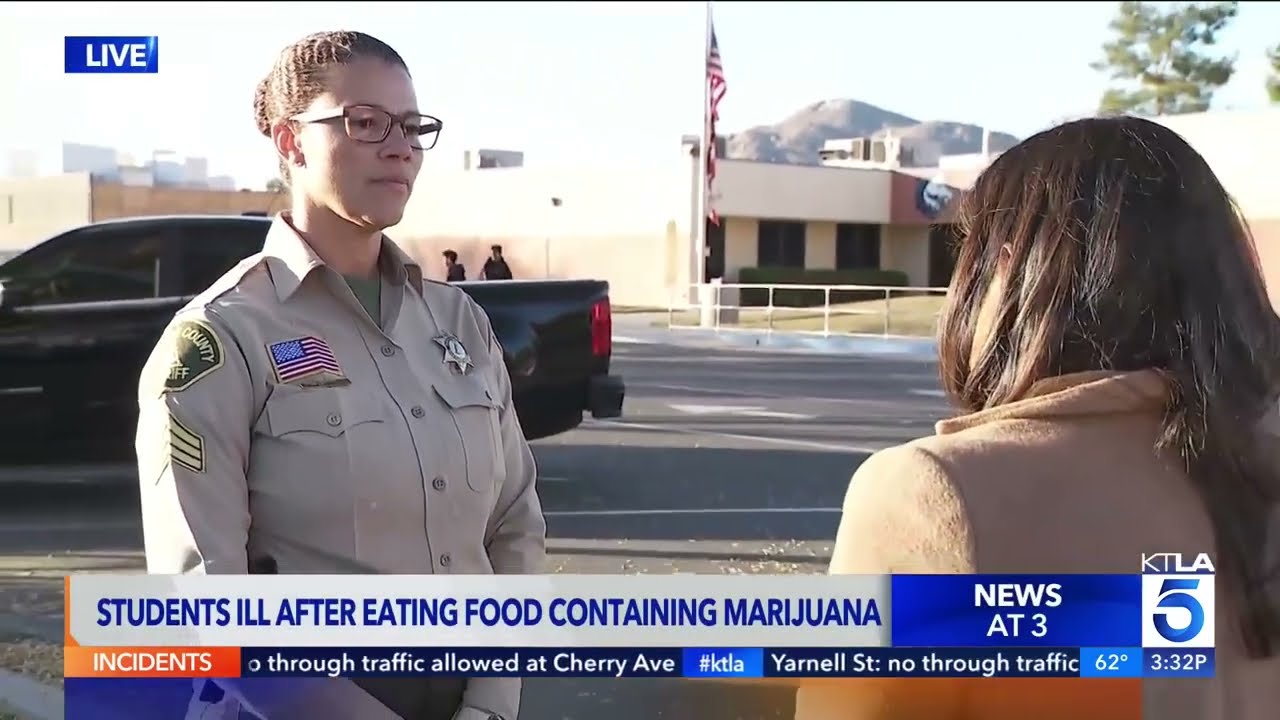The image is a screen grab from a televised news segment, indicated by a news broadcast template at the bottom. In blue writing, it states "Students ill after eating food containing marijuana," followed by "News at 3" in white, and a white square with a blue "5" and "KTLA" above it. There is also a blue rectangle at the top left corner with "live" written in white.

The scene takes place in a parking lot in front of what appears to be an elementary school, identifiable by the building and an American flag in the background. To the left of the image, a female sheriff's deputy is seen. She wears brown-framed glasses and has her hair pulled back in a bun. Her uniform is a tan button-up shirt with a collar, displaying a sheriff's star badge on the left side of her chest and an American flag patch on the right. A black pickup truck, likely a Toyota, is visible behind her. To the right, a woman with long brown hair, presumed to be the reporter, has her back to the camera and appears to be interviewing the officer. The sheriff's deputy is equipped with a gun on her right side and looks calm during the interview.